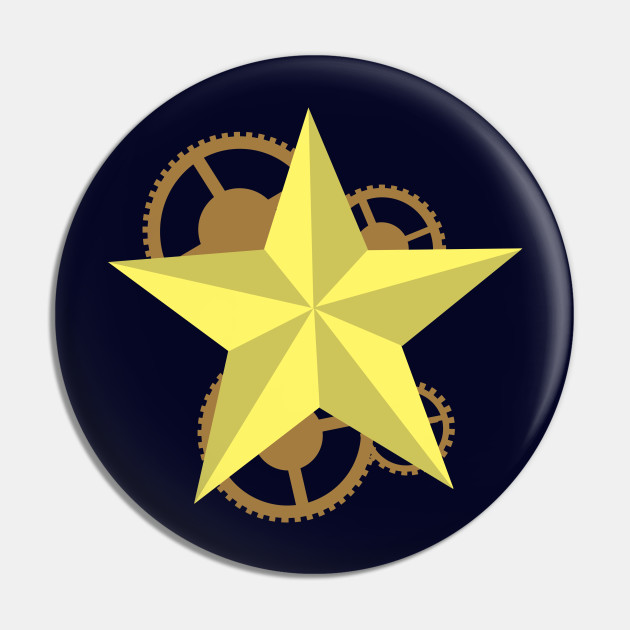The image features a circular badge or button set against a very light gray, almost off-white, background. The badge itself has a dark navy blue or possibly black base, which is overlaid with a prominent five-pointed yellow star at its center. The star is shaded in alternating light yellow and golden yellow tones, giving it a dimensional, 3D effect with the points appearing to be folded. Surrounding the yellow star are four brownish or golden gears of varying sizes laid out on the badge. The largest gear is located in the upper left, followed by the second largest in the lower left, the third largest in the upper right, and the smallest gear in the lower right, resembling the intricate inner workings of a watch. No words or inscriptions are present in the image.